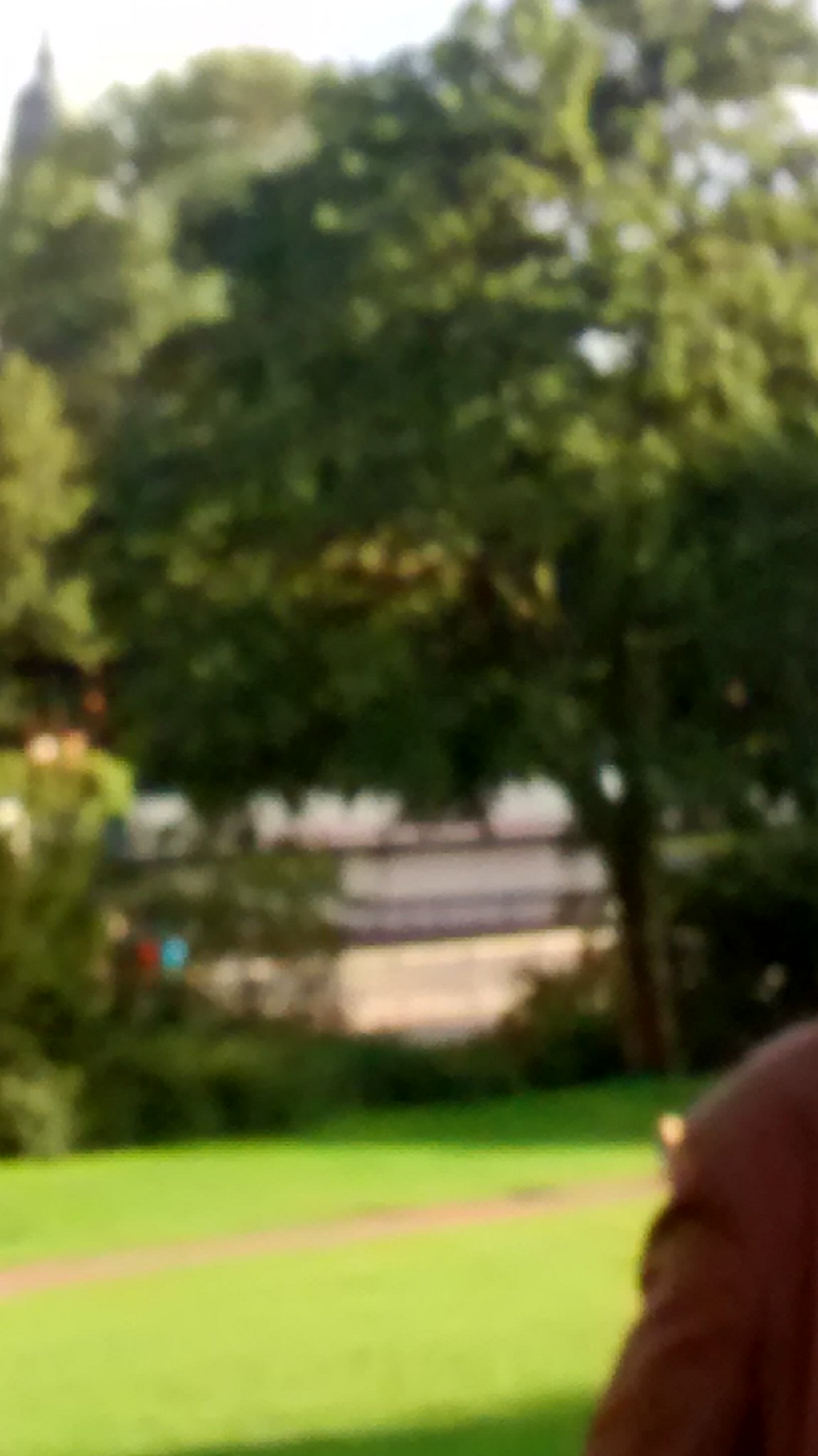The image captures a slightly out-of-focus scene of a park. In the bottom right-hand corner, the shoulder of a person wearing a maroon leather jacket is visible. The foreground features a patch of green grass with a sidewalk intersecting it. Dominating the middle ground is a large tree with abundant green leaves, though the tree's specific type remains unclear due to the focus. Beneath the tree are verdant shrubs, adding layers of greenery to the scene. In the distant background, there appears to be a body of water, hinted at by a bluish patch with straight-lined borders visible just below the foliage of the main tree. A patch of white suggests the presence of a beach.